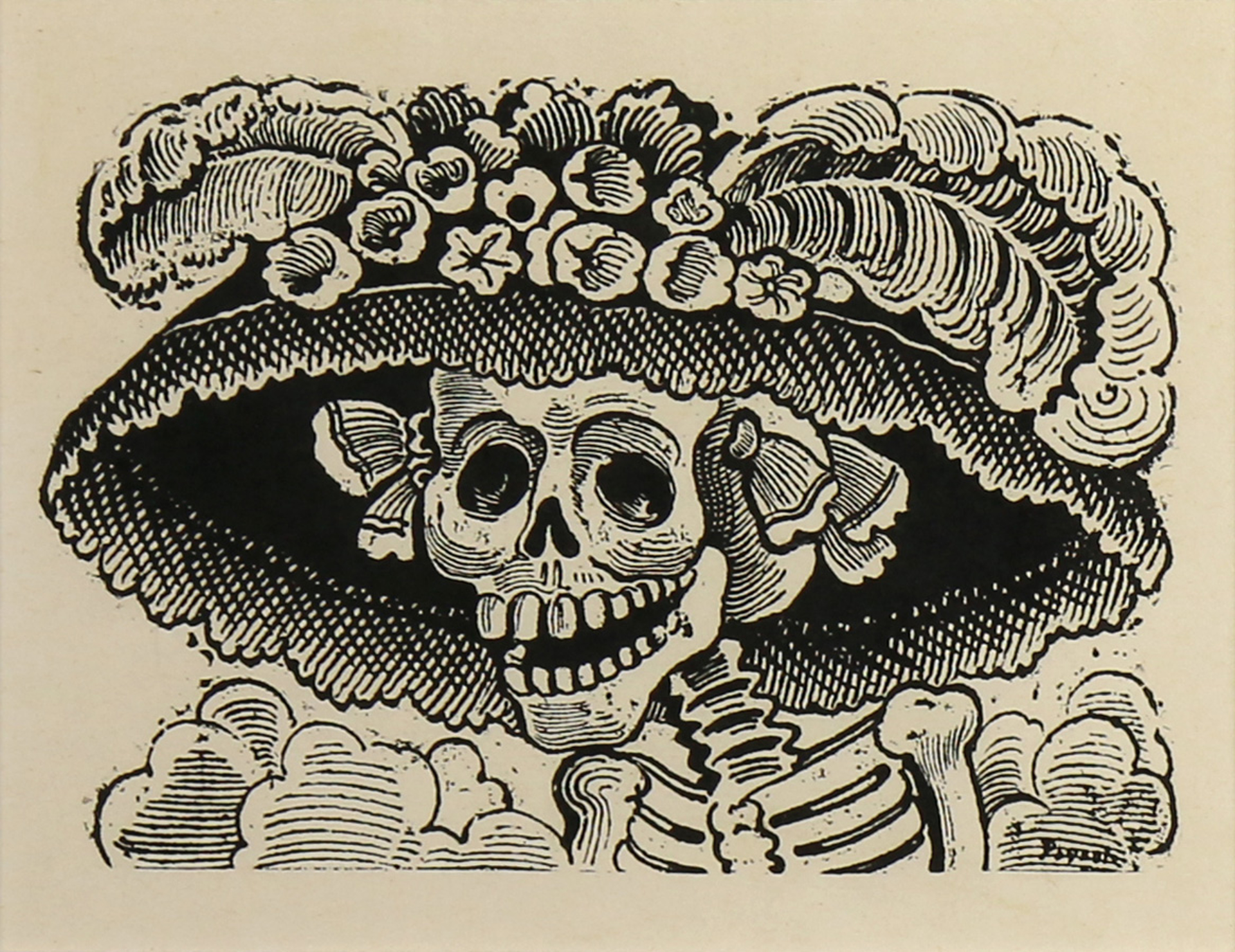This image is a striking and somewhat eerie depiction of a skeleton, executed in black and white on an off-white, tan background. The skeleton appears to be female, characterized by pigtails or ponytails that frame its head. A prominent feature of the skeleton is a large, dome-shaped hat adorned with flowers and two prominent feathers that cascade across the hat's brim, adding an intricate and somewhat ornate touch. The skeleton's mouth is open, revealing very large teeth, and its eyes are depicted as hollow black holes, adding to the macabre atmosphere. Despite being just bones, the skeleton has defined shoulder bones, ribs, and a neck visible. Additionally, smaller round objects are illustrated near each shoulder. There are dark accents used for shading and defining the skeleton, giving depth to the piece. To the left and right of the skeleton, dust clouds seem to emerge, adding to the haunting ambiance. A signature is barely discernible at the bottom right of the image, suggesting the artist’s mark.